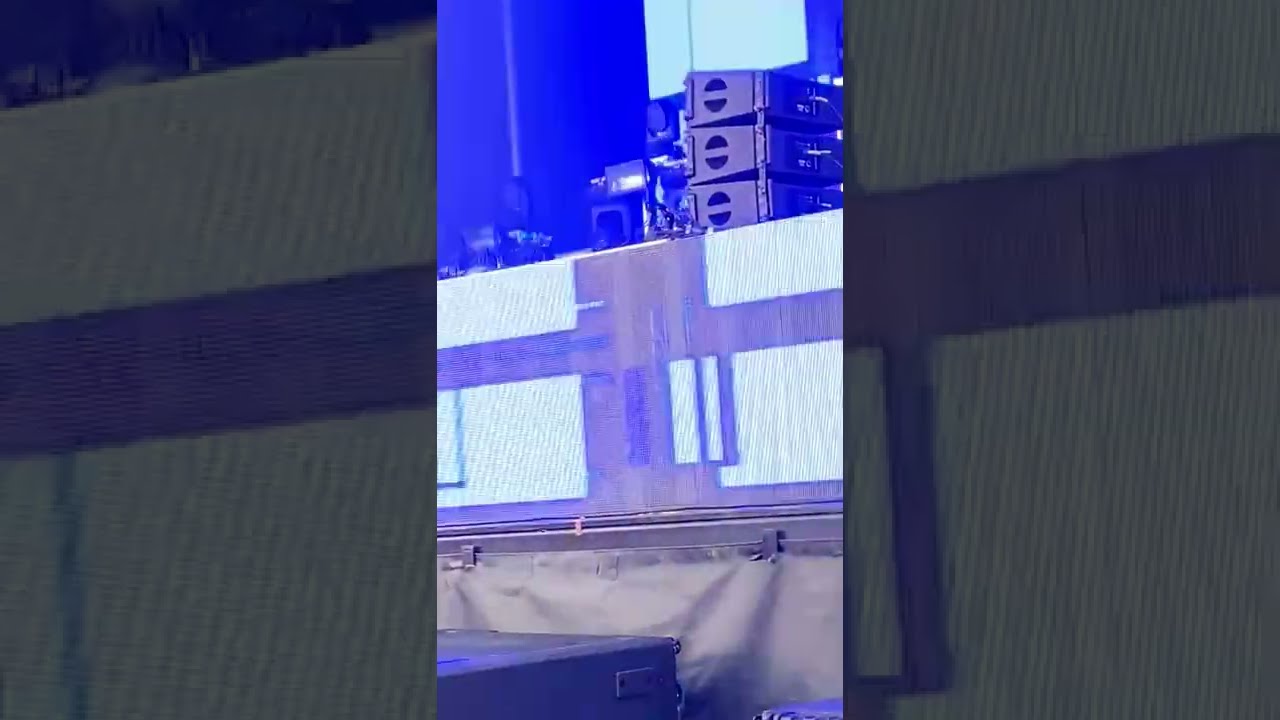The image is a triptych of a concert stage, showcasing both wide and zoomed-in views. The central photograph reveals a tall, metallic crate or box at the bottom, surmounted by a horizontal structure that might be a white tablecloth with designs, suggesting a draped fabric. On top of this setup, three items are stacked along with additional objects to the left. The stage appears tall, around six feet off the ground, and has a gray, possibly rusted appearance, underlined by a black tarp.

Both the left and right images are close-up, darker, and less lit sections of the middle view, emphasizing the borders of the central scene. The overall background is suffused with a bright, light blue illumination, indicating either a light test or ongoing stage adjustments. The setup includes a stack of power amplifiers, likely for guitar, accompanied by various electronic equipment for effects and lighting control. There’s a speaker cabinet barely visible in the bottom corner.

The stage feels expansive and concert-ready, devoid of any people, and dotted with high-tech gear like stacked speakers and a distant large projector screen, possibly prepared for a significant event such as a Taylor Swift concert.